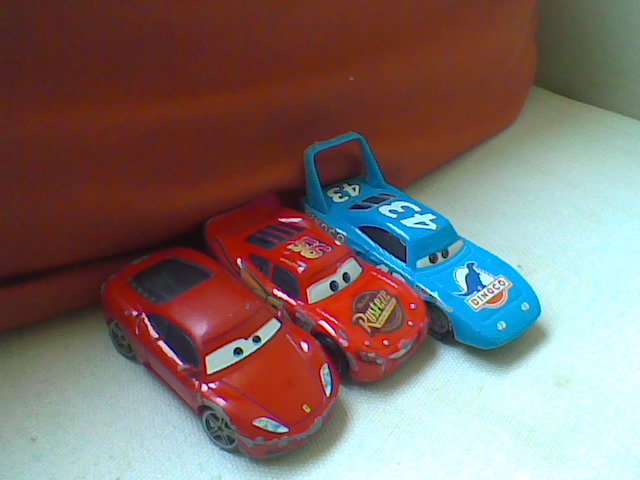This close-up photograph showcases three intricately detailed toy cars from the Pixar movie "Cars," neatly lined up side by side on a gray sofa adorned with a red pillow. The toys, likely die-cast models from a brand like Mattel, appear to be illuminated by overhead lighting, casting subtle shadows and a minor reflection. The leftmost car is a red, Ferrari-like vehicle featuring anthropomorphic eyes on the windshield, giving it an expressive face and a black interior. Prominently displayed in the center is a red race car closely resembling Lightning McQueen, marked with the number 95 on the top and adorned with a Rust-Eze logo on the hood. The rightmost car is a sporty, light blue model branded with the number 43 and the word "Dinoco" on its sleek exterior. These vibrant toy cars stand out vividly against their surroundings, making them an inviting scene for both children's play and collectors' admiration.